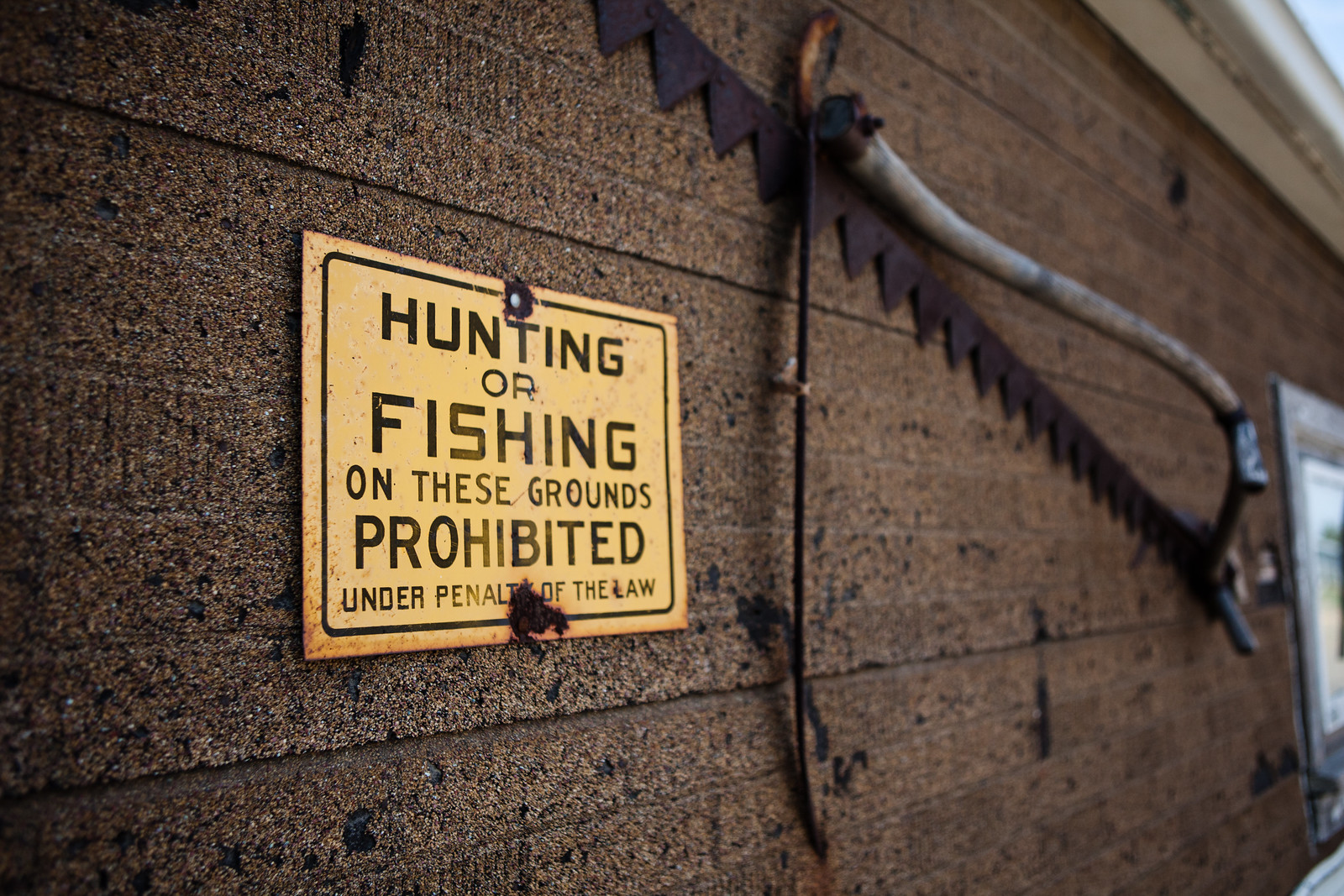The photograph captures a detailed scene of a yellow sign with black lettering, prominently mounted on what appears to be a weathered, brown, wooden wall. The sign, which is just left of center within the frame, reads in bold capital letters: "HUNTING OR FISHING ON THESE GROUNDS PROHIBITED," and in smaller print at the bottom, it states "UNDER PENALTY OF THE LAW." The wall occupies the entire breadth of the image, stretching from the left edge to beyond the right edge, where the top right corner reveals the start of a roof. Adjacent to the sign on the right, an old-fashioned saw is mounted on the wall. This saw features dark, serrated blades and a silver bar over the top that connects to each end, possibly indicating its age and use. The overall setting suggests the exterior of a rustic ranger's office or a similar establishment, evidenced by the presence of a secondary poster or door in the bottom right corner of the frame, and the bright daylight that illuminates the scene.